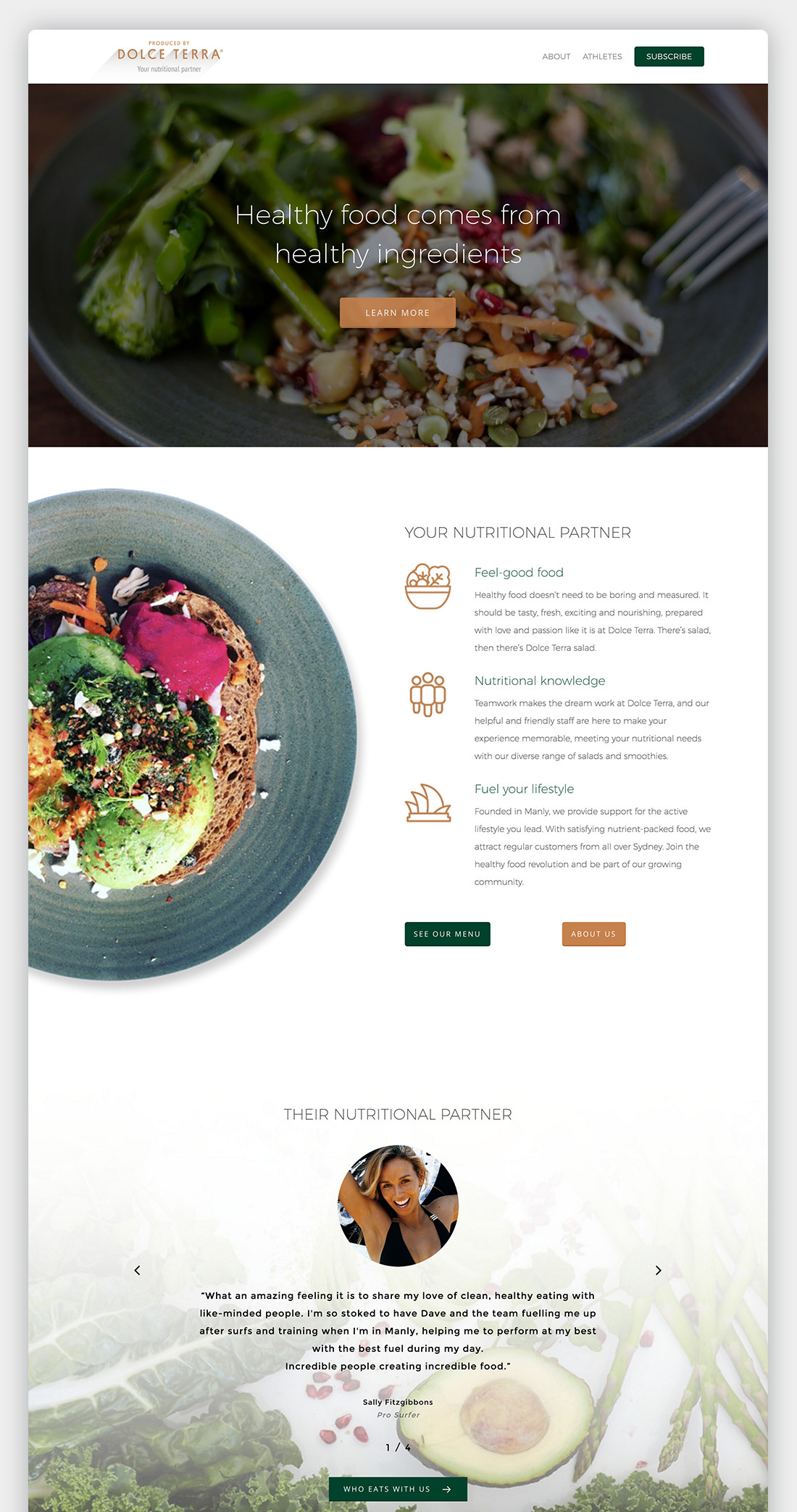On the website for Dolce Terra, a blurred yet intriguing homepage greets visitors. At the top, the slogan "Healthy food comes from healthy ingredients" commands attention, inviting users to click a nearby box for more information. To the left, an appetizing image of a plate of food catches the eye, while to the right, text reads "Your nutritional partners" followed by "Feel good food." Unfortunately, some of the text beneath these headings is too indistinct to decipher. Lower down, the terms "Nutritional knowledge" and "Feel your lifestyle" stand out, again accompanied by unreadable text. Two clickable options appear below this section, titled "About Us" and an unclear second choice. The tagline "Their nutritional partner" introduces a circular photo of a smiling young Caucasian woman in a bathing suit. Below her image, a quote seems to express the founder's joy in sharing a passion for clean, healthy living with like-minded individuals, though the exact wording is obscured.